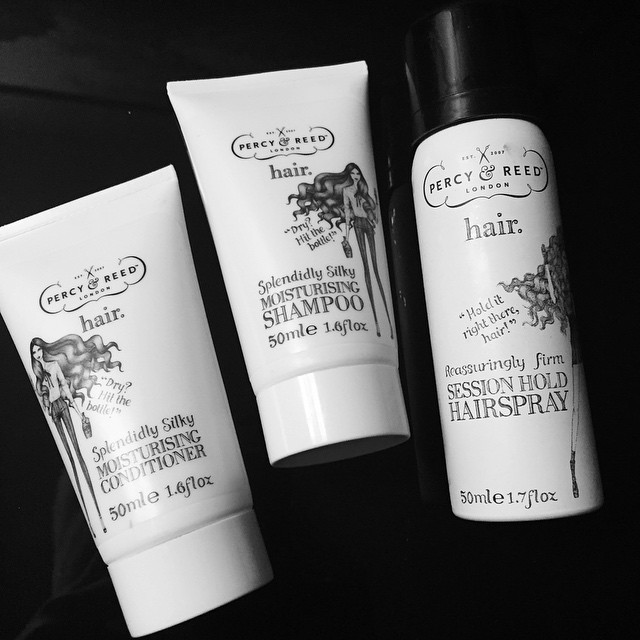In this image, three hair care products from the Percy Reid London collection are prominently displayed against a solid black background. Positioned centrally, these items exude a sleek and unified aesthetic with their monochromatic color scheme comprising black, white, and various shades of gray. On the left, we find the "Percy Reid Hair Splendidly Silky Moisturizing Conditioner" bottle. In the center, the "Percy Reid Hair Splendidly Silky Moisturizing Shampoo" bottle takes focus. Finally, on the right, the "Percy Reid London Hair Reassuringly Firm Session Hold Hairspray" completes the trio. The layout and styling suggest that this could be a professional stock image, ideal for use on a hair care website or in a polished advertisement.